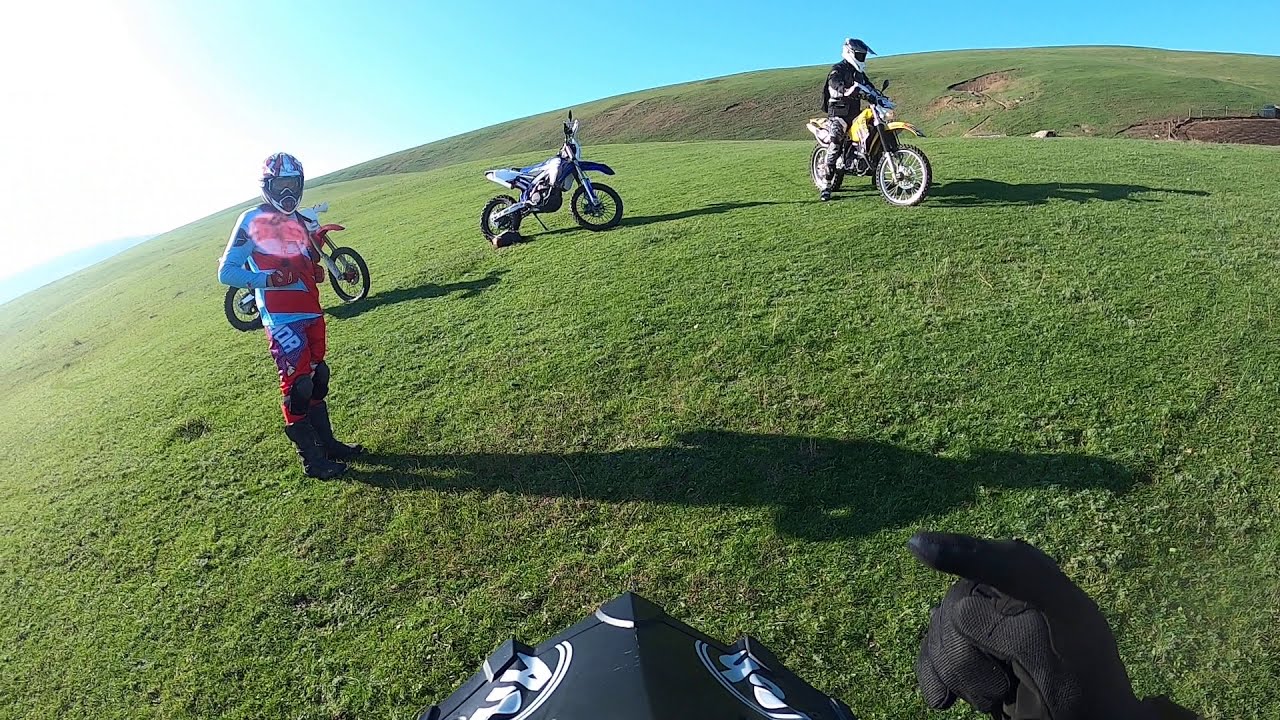In this vibrant outdoor photograph, a vast, hilly grass field stretches out under a brilliant blue sky. The undulating terrain is alive with lush green grass, bathed in strong sunlight emanating from the top left corner, casting long shadows of the subjects onto the ground. At the center of the image, three motorcycles are strategically positioned. Two of the bikes remain unoccupied, while the third, a yellow motorcycle, has a rider clad in a black jacket and helmet, actively astride it. Nearby, another rider, dressed in a striking blue and red motorcycle jacket with knee pads and black boots, stands on the ground looking directly at the viewers with his white helmet gleaming. To the left, another rider in a white and red suit with black boots adds to the lively assembly. The perspective reveals the rider's gloved hand at the bottom of the image, pointing towards the group, capturing a dynamic moment of camaraderie amidst the serene and expansive grass field.